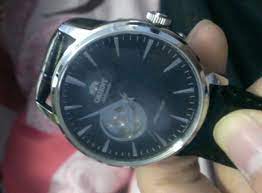In this image, a person is holding a sophisticated wristwatch with a black leather band. The watch is angled so that the top portion appears on the left and the bottom portion on the right. The timepiece features a sleek, black face with silver accents, including silver markers in place of numerals. Adding a touch of luxury, the center of the watch face contains a circular design that seems to be embellished with sparkling stones, possibly diamonds or crystals. The holder's thumb is visible resting on the upper part of the band, while another finger supports the bottom. The blurred background suggests the presence of fabric or clothing, adding a textured backdrop to the detailed foreground of the elegant watch and hand.